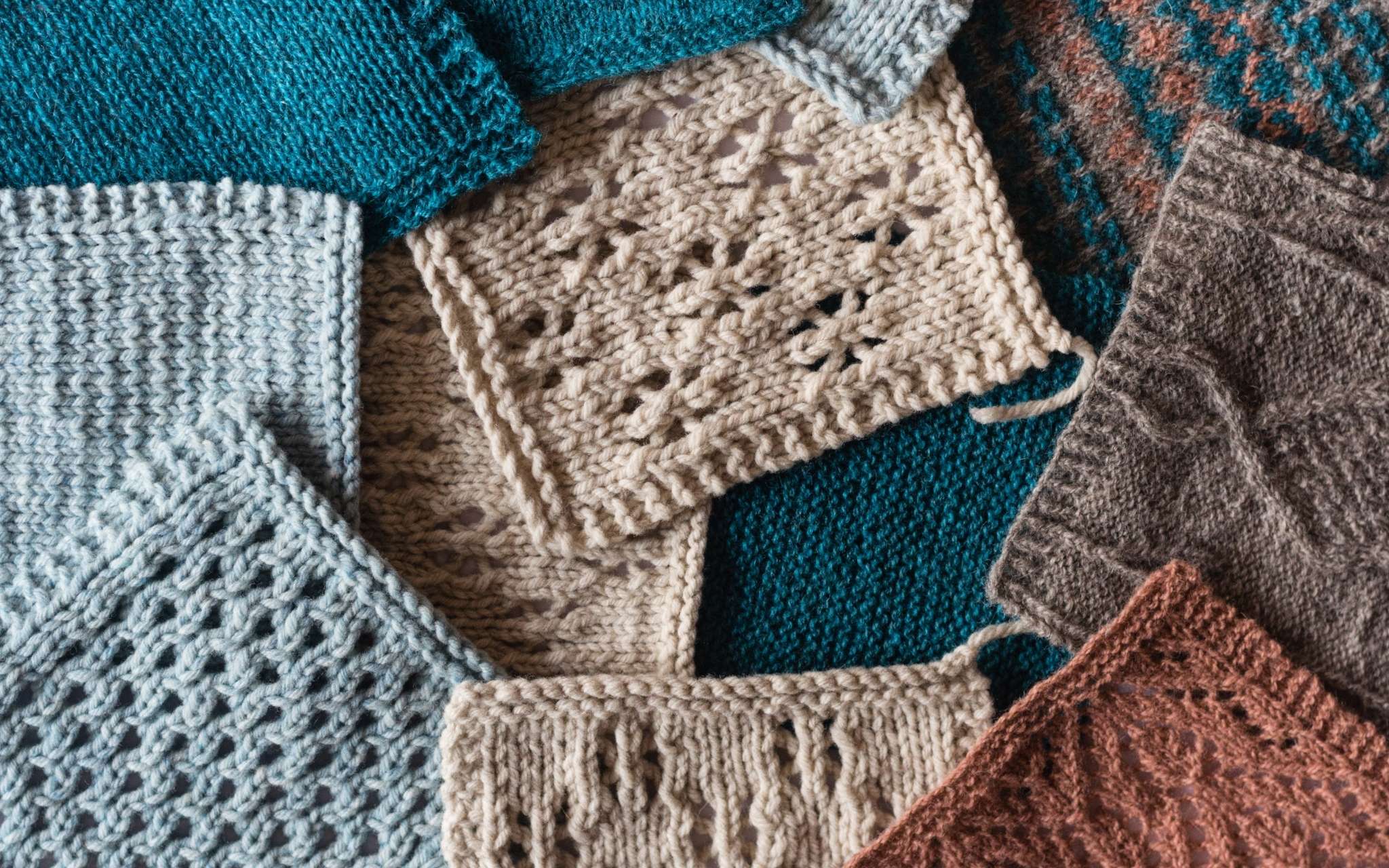The image features an assortment of small, square-shaped pieces of knitted cloth, resembling coasters or placemats, made from yarn material. They are scattered around and lie in a pile, partially overlapping each other, exposing only portions of their vibrant array of colors. Among the notable hues, you can see green at the top, light blue on the left, tan in the middle, and darker brown on the right, along with some baby blue, turquoise, blue-green, beige, grayish-brown, and a hint of reddish-orange at the bottom. Some pieces have strings dangling from their corners, while others showcase delicate stitched patterns, including shapes reminiscent of snowflakes and bells, with uniform holes scattered across some pieces. In total, there appear to be about 12 of these cloths, each contributing to the rich, colorful tapestry of the scene.